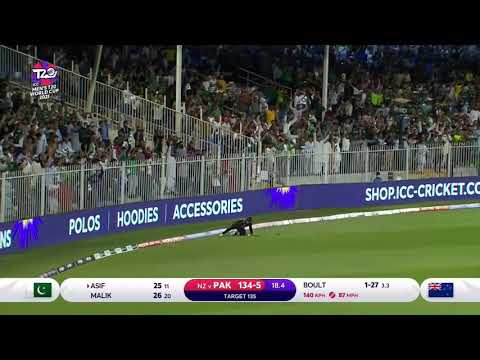This color photograph captures a moment from a cricket match in a sports stadium, likely a screen grab from a replay. At the center of the image, a player dressed in black is on their hands and knees on the green astroturf field. The upper third of the image shows a high white metal fence holding back the crowd, with hundreds of spectators visible in the bleachers. Advertisements for "shop.icc-cricket.com" featuring polos, hoodies, and accessories appear prominently on a blue background around the field. The upper left corner bears a television channel logo. Along the bottom edge, there's a white border and team statistics displayed in text, including a black box with a red line and a purple line. The text within the box reads "ASIF 2515 AM ALIK 2620," while the score on the right side indicates "PAK 134-5". The image offers a vibrant and detailed view of the stadium’s atmosphere, with fans holding signs and columns interspersed among the seated crowd.